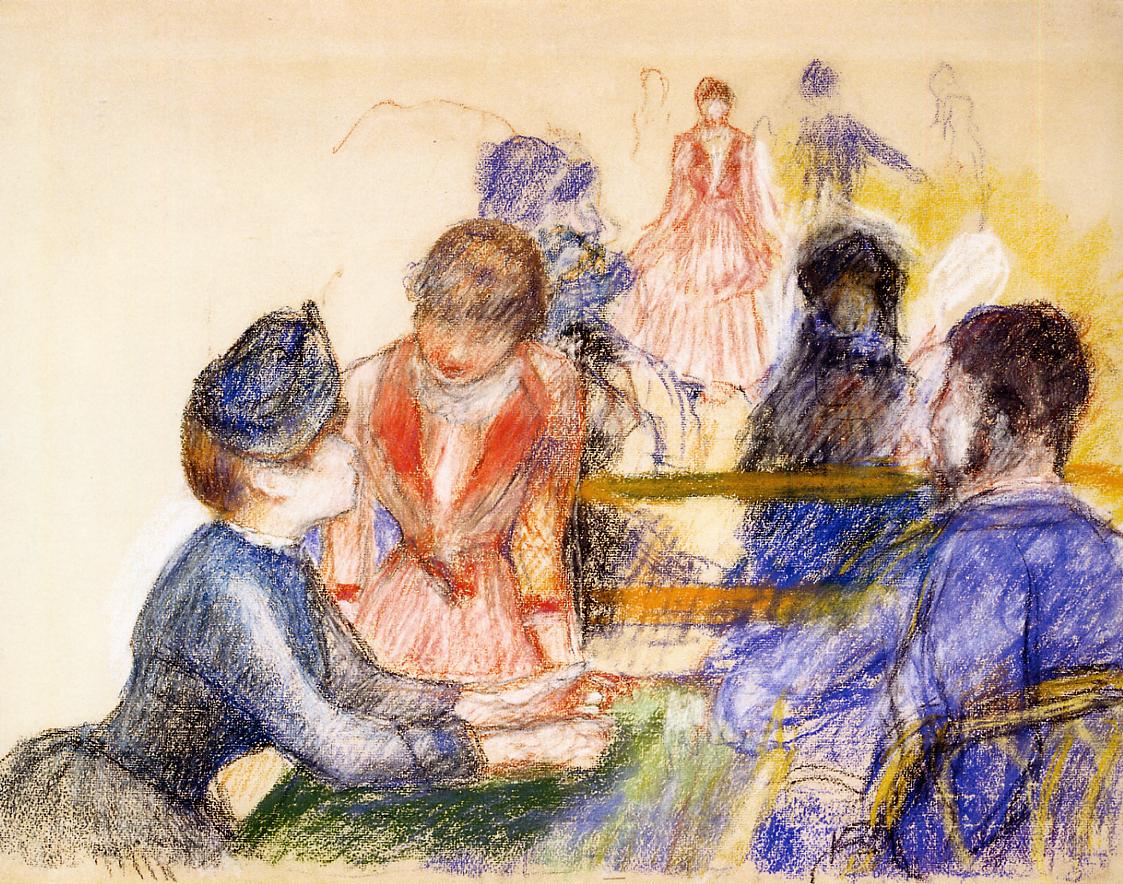The image is a detailed and colorful depiction, likely created with chalk or crayon, of a lively 18th or 19th-century gathering. Central to the composition is a table where three people are seated in the foreground: a young lady on the left, dressed in a large dress with a bonnet, talking to another young lady. A man with a beard, possibly in a uniform, sits across from them. The vivid scene suggests an outdoor setting, perhaps at a restaurant, indicated by the fence separating the table from the background. Behind the primary figures, several more people—four distinct individuals—can be seen standing or moving around, possibly dancing. The figures in the background, adorned in blue and rose-colored outfits, contrast against the minimalist white space and faint yellow outlines that frame the scene. The image combines a blend of incomplete outlines and defined characters, creating a nostalgic and historical ambiance.